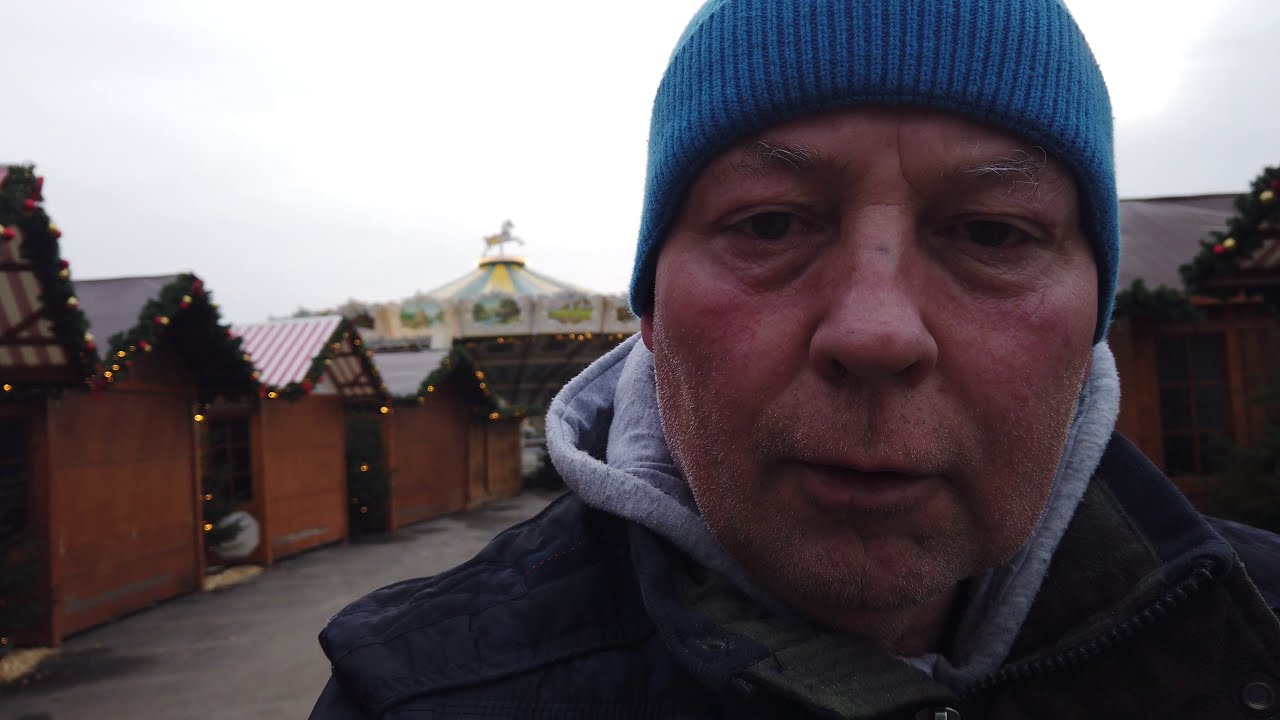In this detailed color photograph, a close-up captures a bundled man standing in a cold, festive plaza. He is around 50 or 60 years old, wearing a blue knit beanie, a gray hoodie beneath a dark blue jacket with a green collar. His face is slightly red with rosy cheeks and a bit of scruff, as if he has a five o'clock shadow. His mouth is slightly open, giving the impression he is about to speak. The man stands prominently in the right side of the image.

The backdrop features a row of small, triangular-roofed shops, likely storage sheds or business stalls. Each shop is adorned with Christmas decorations, including garlands made of pine or evergreen and lights along the roof edges. Four shops are visible, appearing closed with boards across their fronts. In the distance, a decorated carousel with a horse figure on top adds a whimsical touch to the scene. The sky above is overcast, hinting at a cold, wintry day, enhancing the festive yet chilly atmosphere of the photograph.